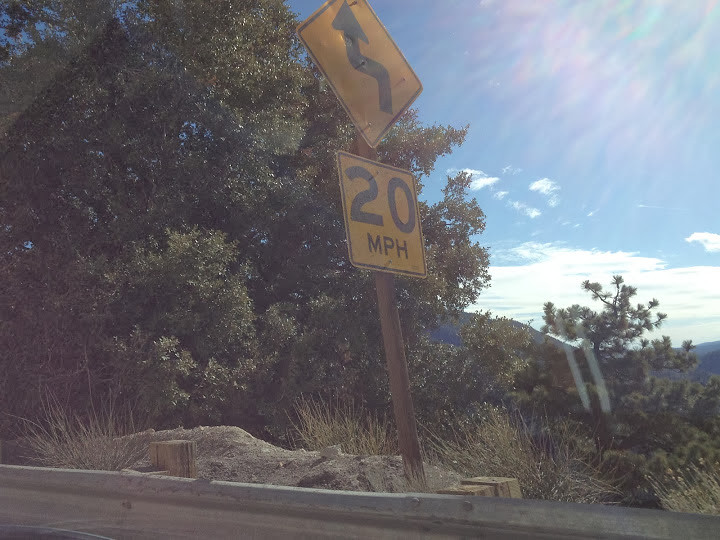The image depicts a detailed roadside scene. At the forefront, a road sign is prominently featured, consisting of two parts: a lower square-shaped sign with a yellow background displaying "20 MPH" in black lettering, and an upper diamond-shaped sign with a black arrow indicating a winding road ahead, also set against a yellow background. Both signs are mounted on a gray metal pole anchored in the ground. In front of the pole, a gray highway railing runs horizontally, supported by brown wooden stakes for reinforcement. Behind the road sign, a rugged landscape unfolds with a mixture of rocky terrain, brown and green foliage, and scattered plants resembling straw. The background is graced with green trees, and further back, mountainous formations loom in the distance. The sky above is a vibrant blue, scattered with white clouds that grow denser towards the horizon, with a wisp of multicolored light—white, purplish, and a hint of blue-green—emanating from the upper right, indicative of the sun's position.